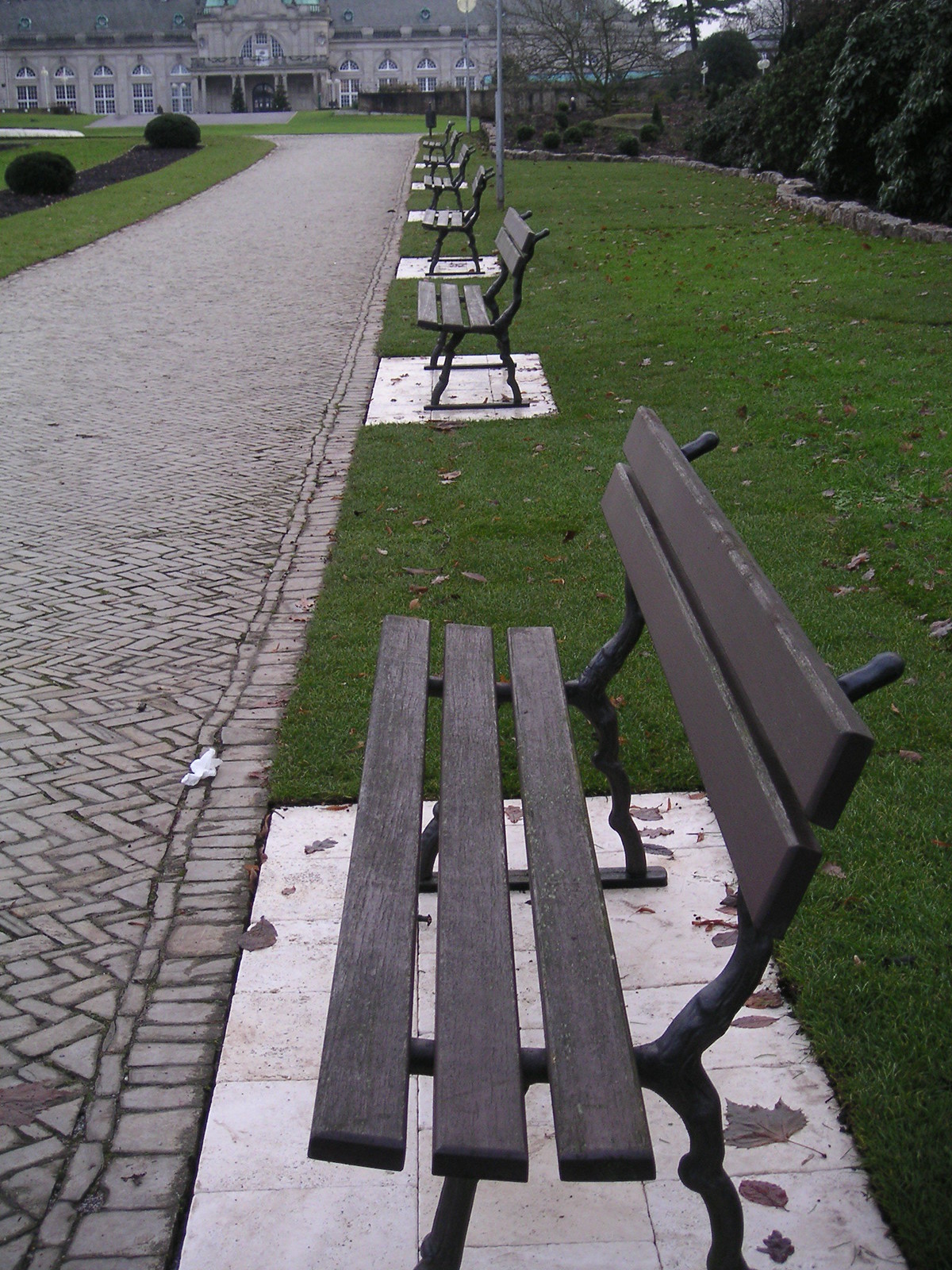The image portrays a serene outdoor setting in a park or the garden of a grand mansion, with a portrait orientation. Six neatly aligned gray benches with distinct black, rigid metal frameworks are positioned along a path made of stone arranged in a zigzag pattern. Each bench features two long baseboards for the back and three baseboards for seating. These benches rest on small concrete slabs amidst lush green grass. 

To the left of the benches, the intricate stone path meanders, while the backdrop on the right is defined by tall hedges. The landscape includes various trees and rocks, contributing to the picturesque scenery. In the distance, a magnificent gray mansion looms, featuring a central entrance adorned with a balcony. Above the entrance, a unique window—either triangular or semicircular in shape—crowns a standard rectangular window with four panes. The mansion, almost reminiscent of a castle with its impressive size and stone façade, adds a touch of grandeur to the tranquil park setting.